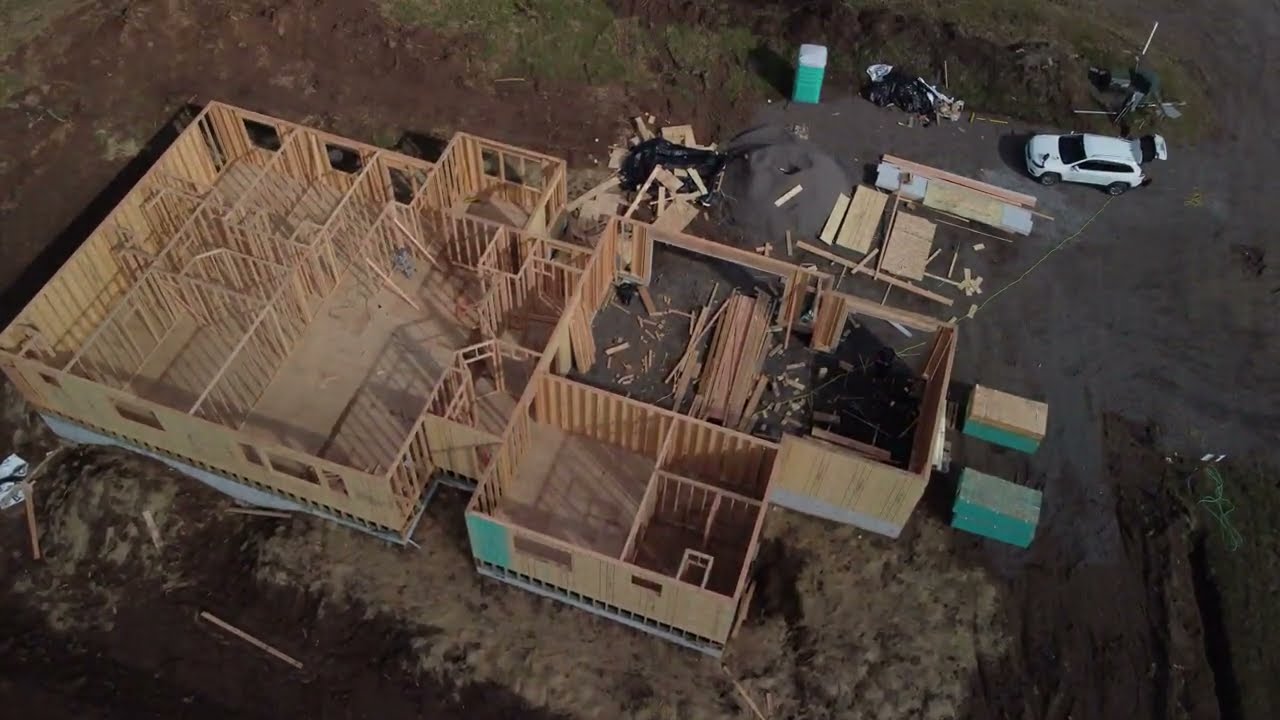This overhead drone shot showcases a house under construction. The building, with its light brown wood framing and exposed floor plan, lacks a roof, revealing various rooms outlined by two-by-fours. The structure is surrounded by a vast, disturbed brown dirt area with no visible grass, indicating ongoing construction work. Notable elements include stacks of lumber and building supplies, positioned around and within the structure. A white car, possibly an SUV with its trunk open, is parked in the top right corner of the image. Additionally, a green and white porta potty is situated towards the top middle of the scene. The overall image emphasizes the early stages of construction, marked by an open foundation and numerous construction materials scattered around the site.